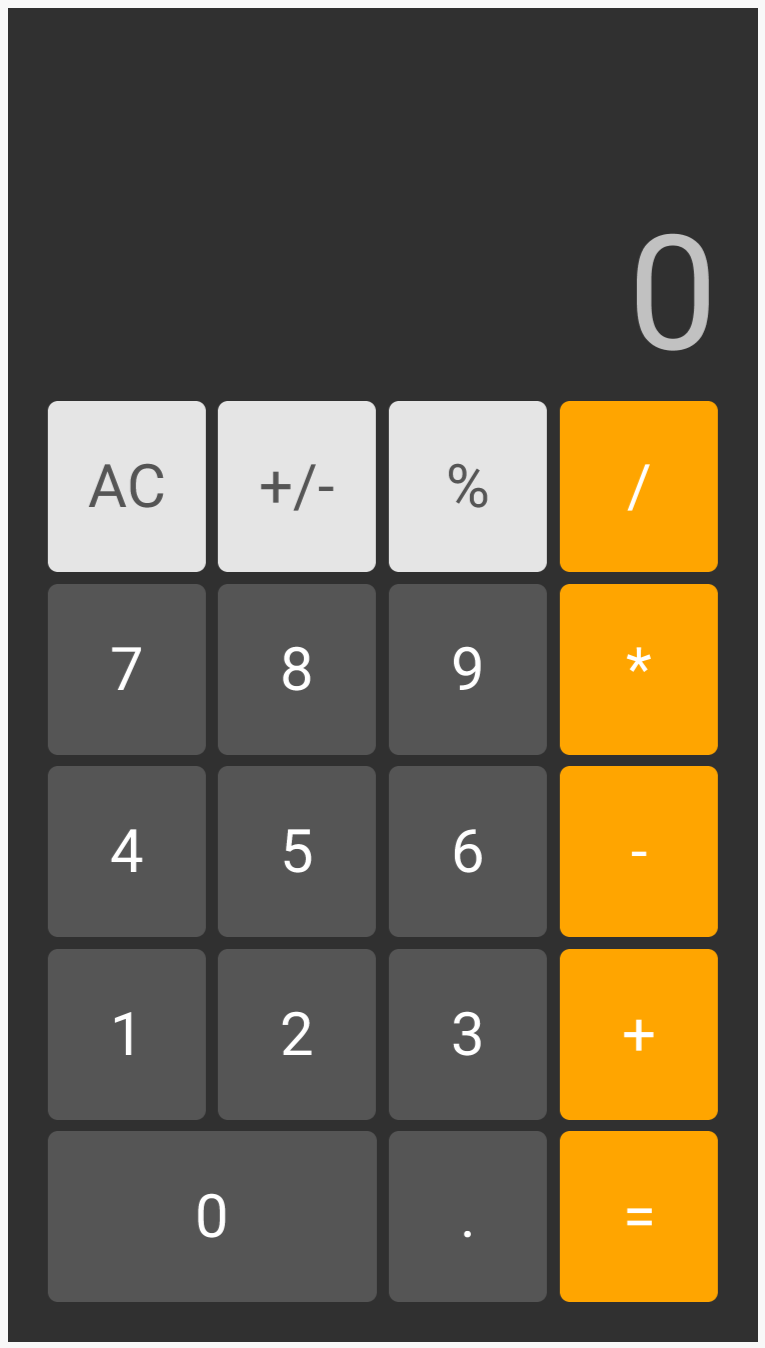The image is a digital screenshot of a calculator app with a meticulously organized interface against a very dark grey background. The numbers are displayed in semi-dark grey tones, creating a subtle yet visually coherent design. Across the top row, from left to right, are three function buttons set against a lighter grey background: "AC," indicating the clear function, "+/−" for changing the sign of the entered number, and "%" for percentage calculations. 

On the right-hand side of the app, vertically aligned, are five function symbols with an orange background: from top to bottom, these are the division sign ("/"), multiplication sign ("*"), subtraction sign ("-"), addition sign ("+"), and the equals sign ("="). 

A grey zero is positioned at the top right, just above the beginning of the keypad. The keypad consists of 19 square buttons in total. Directly below the top function row are the numerical buttons and additional function keys: 

- The second row features the numbers 7, 8, and 9, all in a dark grey background.
- Adjacent to these numbers, in an orange background, is the multiplication sign ("*").
  
The third row follows with the numbers 4, 5, and 6 against a dark grey background, accompanied by the subtraction sign ("-") on an orange background.

In the fourth row, we see the numbers 1, 2, and 3 on a dark grey background. Next to them is the addition sign ("+") with an orange background.

The bottom row contains a long rectangular key featuring the number 0, evenly spanning the width of the buttons for numbers 1 and 2. This is followed by a decimal point (".") button in a dark grey background and the equals sign ("=") button in orange.

Currently, the calculator app displays no active calculations, effectively showing a blank slate ready for input.